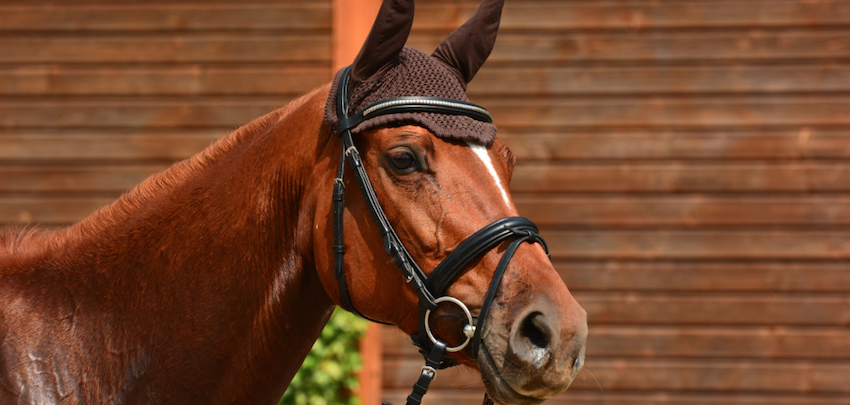This image showcases a chestnut brown horse with a deep chestnut coat. The focal point of the picture is the horse's head and neck, adorned with a white stripe running from its forehead to its nose, between its eyes. The horse wears a woven cap that covers its ears and part of its head, under a black bridle featuring a circular silver ring. The mane appears brushed to one side, sharing the same rich chestnut hue as its coat. Notable veins are visible on its face, emphasizing its healthy physique. Captured on a bright, sunny day, the scene is set against a backdrop of horizontal dark brown wooden paneling, with a hint of green shrub visible beneath the horse's neck. The horse stands facing the right side of the frame, appearing calm and poised.